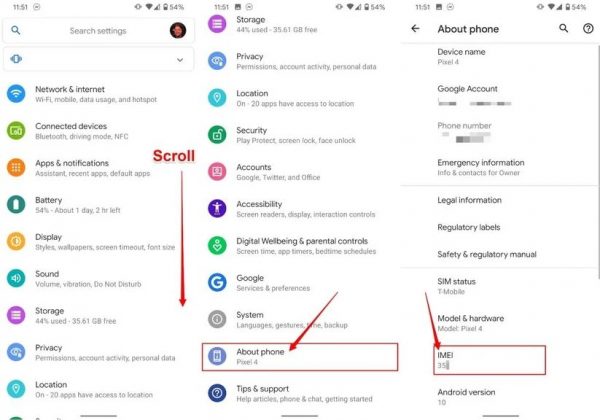This image features three screenshots of a smartphone settings menu, each with specific annotations. Across all screenshots, the top bar displays a consistent status: the time reads 11:51, there is a vibration icon, full Wi-Fi signal, three bars of cellular signal, and the battery charge at 54%.

The first screenshot shows the "Search settings" menu. On the top right, there's a user's photo within a circular frame, and a search magnifying glass icon is on the top left. Below this, an icon likely indicating vibration mode and a downward arrow are visible. Various settings options are listed with circular icons in different colors on the left side, including "Network and internet," "Connected devices," "Apps," "Notifications," "Battery," "Display," "Sound," "Storage," "Privacy," and "Location." A red text annotation with an arrow suggests scrolling down.

The second screenshot continues the list, displaying "Storage," "Privacy," "Location," "Security," "Accounts," "Accessibility," "Digital Wellbeing and parental controls," "Google," "System," "About phone," and "Tips and support." The "About phone" option has a red arrow pointing towards it, and a red rectangle surrounds the "About phone" option.

The third screenshot details the "About phone" section for a Pixel 4. Visible information includes the device name "Pixel 4," a Google account (with details pixelated out for privacy), and the phone number (also pixelated). Other entries listed are "Emergency information," "Legal information," "Regulatory labels," "Safety and regulatory manual," "SIM status," "Model hardware," and a partially pixelated IMEI number starting with "35". This section is bracketed by a red rectangle and marked with a large, swooping red arrow for emphasis.